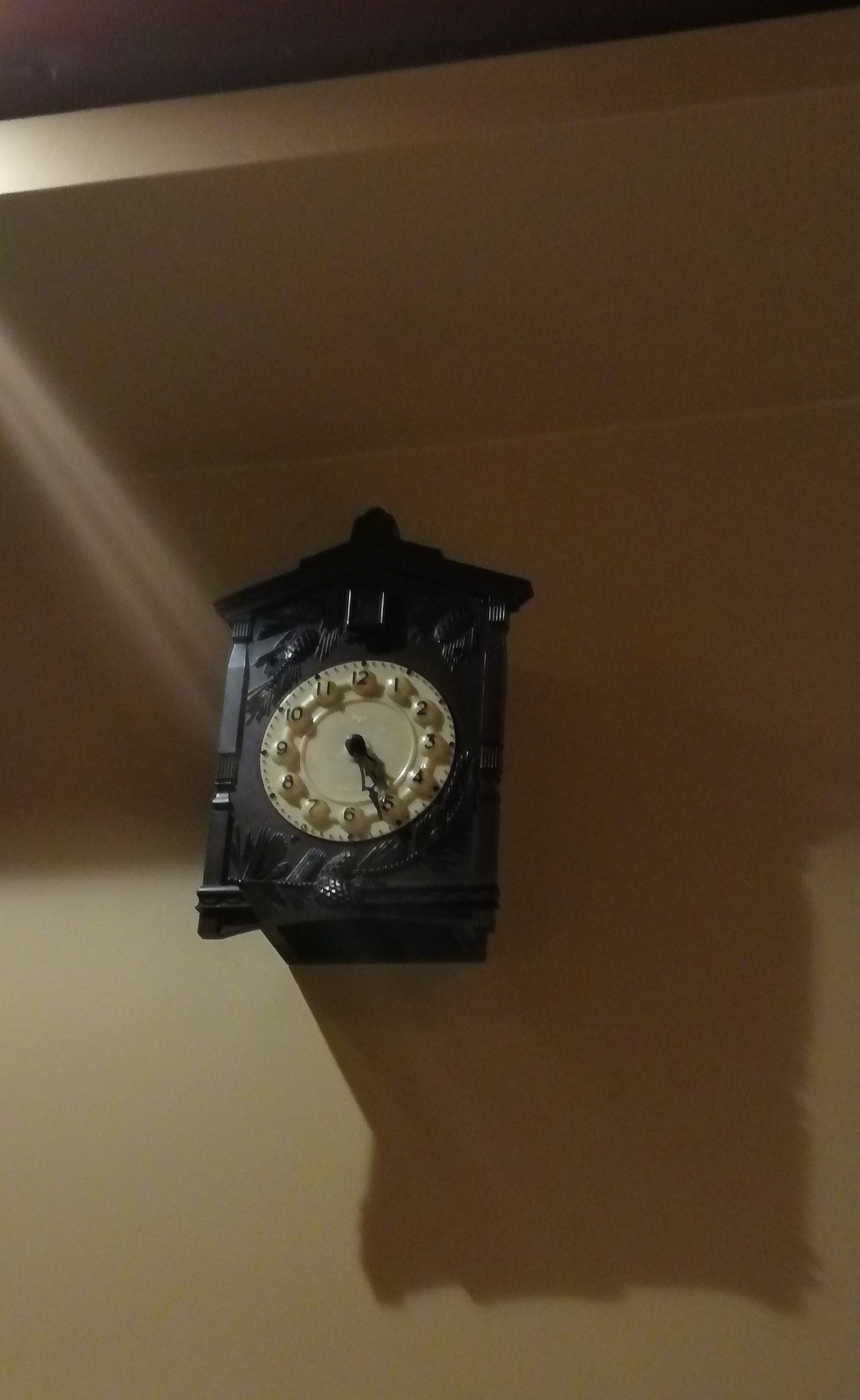"An intricately designed black cuckoo clock stands prominently against a tan-colored wall, its craftsmanship reflecting a classic and timeless appeal. The clock features a white face with black Arabic numerals, each number encased in a spherical shape connected by a circular band, adding a unique three-dimensional element. The hour and minute hands exhibit an elegant, vintage design with curved, pointed tips and cut-out interiors, accentuated by two supporting pieces and a thickened end. Notably, the minute hand draws the most attention with its refined detailing.

Surrounding the clock face are ticks marking the minutes, with every five-minute increment distinguished by a thicker tick. The body of the clock resembles a rectangular box crowned with a gabled roof that boasts a prominent, wide ridge. Decorative elements, perhaps inspired by plant life, adorn the clock, gracefully wrapping around the lower and upper sections.

The top of the clock features a small, subtly opened door positioned just below the roof's peak and above the numeral 12. Though no figure is visible, the tiny, dark door contrasts sharply with the bright faceplate beneath it. The clock is meticulously crafted with elements of black and brown hues, which are most apparent in the upper left corner of the image, providing a rich contrast against the background wall. The sophisticated blend of colors and the detailed design elements evoke a sense of timeless elegance and meticulous craftsmanship."